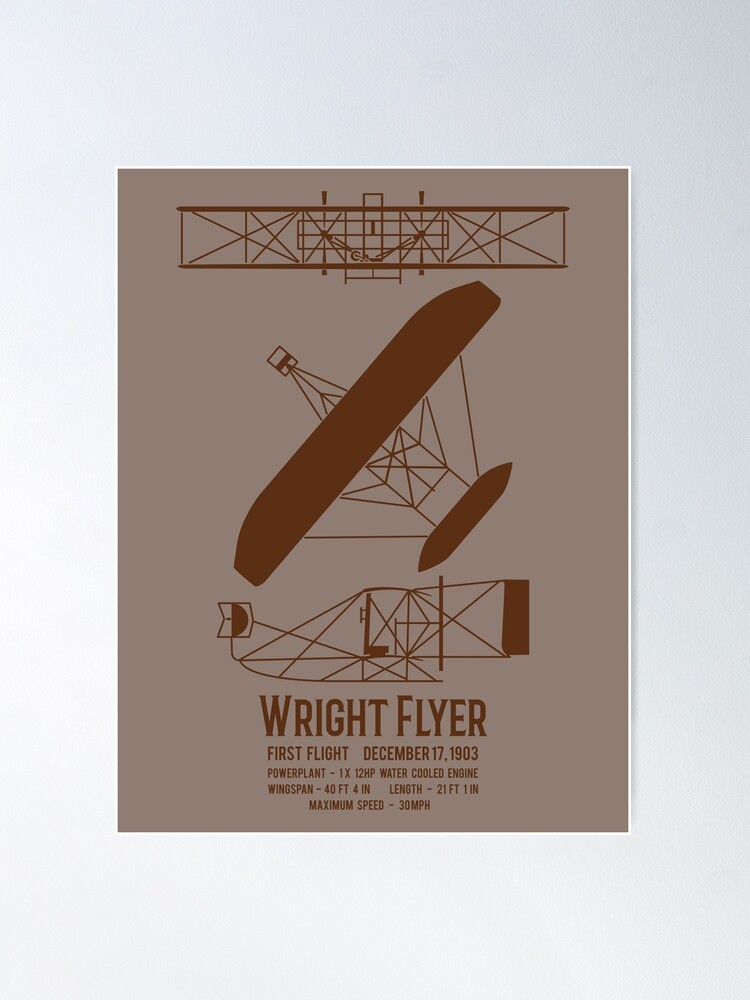This poster features a finely detailed, line-drawn image of the Wright Flyer, the pioneering airplane designed by the Wright brothers. Displayed against a light gray background, the poster itself is rendered in tan and darker tan tones, lending it a monotone yet historically reverent aesthetic. The careful line art illustrates the intricate structural engineering of the airplane, capturing its wingspan and the hub of the plane with precise geometric lines. 

Text at the bottom of the poster provides detailed specifications of the Wright Flyer: "First Flight, December 17th, 1903," followed by "Power Plant: 1X, 12 HP Water-Cooled Engine," "Wingspan: 40 feet 4 inches," "Length: 21 feet 1 inch," and "Maximum Speed: 30 MPH." This poster, hanging vertically, depicts three different angles of the aircraft, offering an insightful visual representation of this landmark in aviation history.